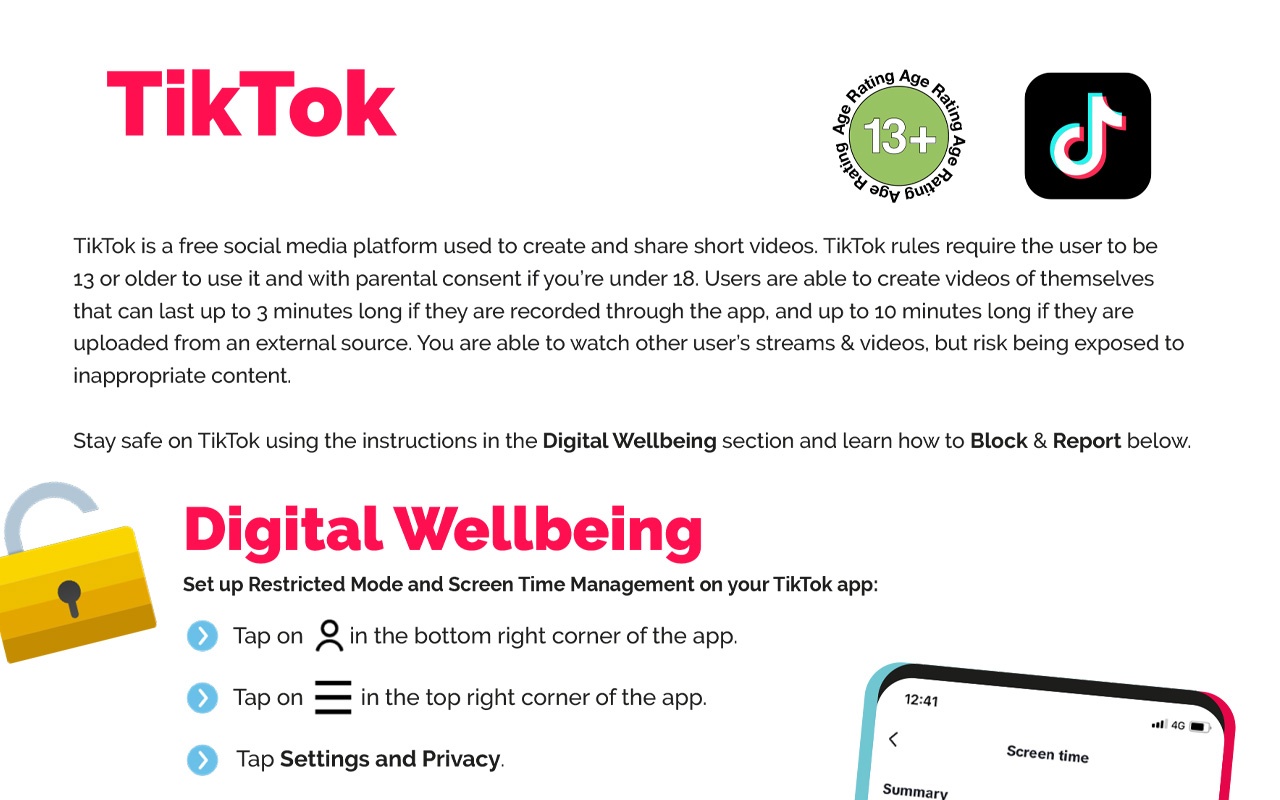**Caption:**

This image illustrates safety guidelines and settings for TikTok users, emphasizing the platform's digital well-being features. TikTok, a free social media platform known for its short video content, mandates that users be at least 13 years old and requires parental consent for users under 18. Videos created within the app have a maximum length of three minutes, while externally uploaded videos can be up to ten minutes long. 

The main focus of the image is a section dedicated to staying safe on TikTok. It provides instructions for setting up restricted mode and screen time management, aimed at minimizing exposure to inappropriate content. A padlock icon represents security and digital well-being, bolstering the message of online safety. The instructions detail which buttons to tap within the app to adjust these settings.

The image features a clean design with a white background and black text, accented with red elements for emphasis. The TikTok logo appears on the top right alongside an age restriction note indicating "13+." In the bottom right corner, there's a depiction of a smartphone displaying TikTok settings, reinforcing the instructions on managing safety features effectively.